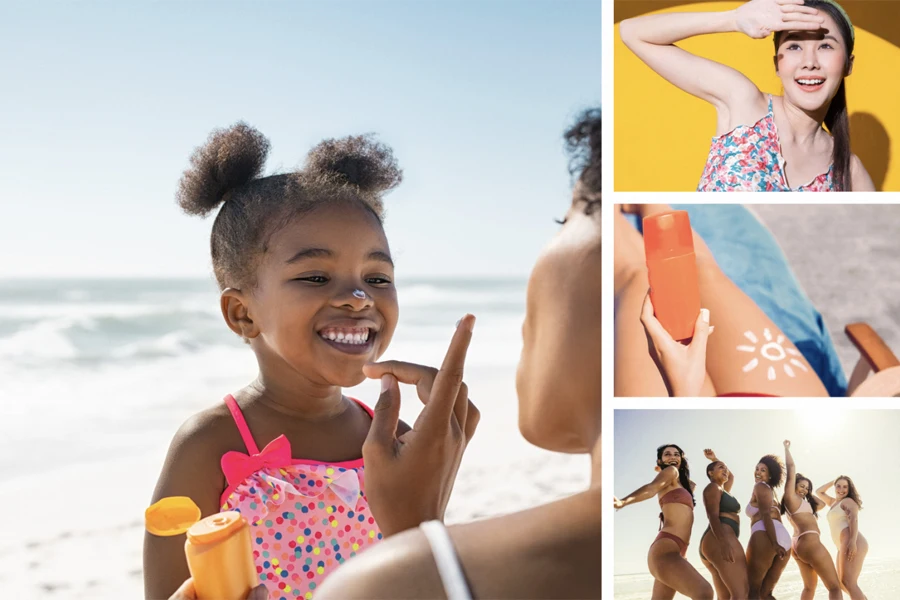The image is a collage of four separate photos, with the largest photo on the left and three smaller photos stacked vertically on the right. The main photo features a black-skinned mother and her smiling young daughter at the beach. The mother, holding a yellow bottle of sunscreen, is applying it to the child’s nose, which has a small dollop of sunscreen. The daughter, dressed in a pink swimsuit with multicolored polka dots and two little pigtails on top of her head, appears delighted. The beach setting includes sand and distant waves.

On the right, the top photo shows an Asian or mixed-descent girl with long black hair, wearing a floral tank top or bikini top against a bright yellow background. She is shielding her eyes from the sun with her right hand, casting a shadow on her face.

The middle photo depicts the legs and hand of a woman seated, possibly poolside. In her hand, she holds an orange bottle, likely sunscreen, while a crude sun design made of sunscreen is drawn on her leg.

The bottom photo captures five women dancing at the beach, each wearing a different colored bikini—maroon, green, lilac, light pink, and light yellow—adding to the vibrant, sunny beach atmosphere.